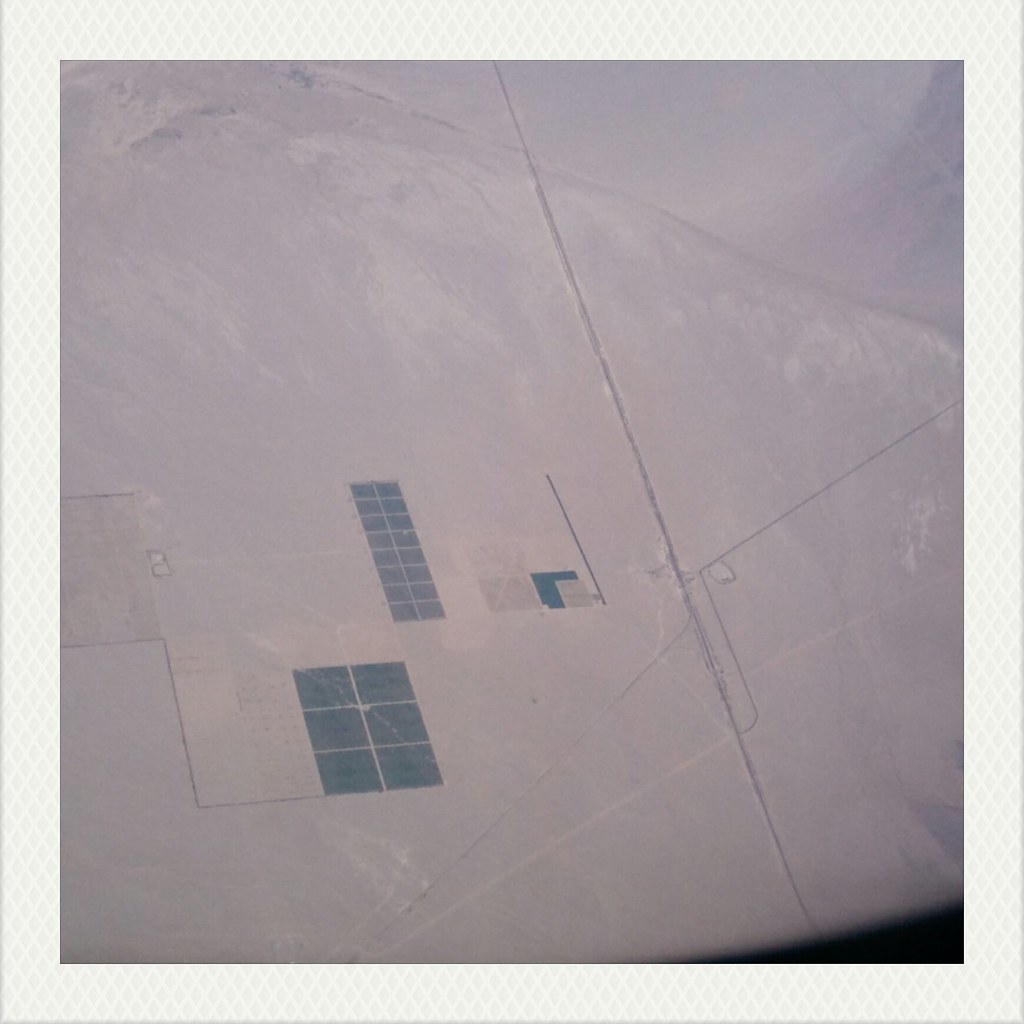This image features an abstract, crumpled piece of white or light gray plastic or paper, occupying the majority of the frame except for a small black section in the bottom right corner. A series of lines and shapes create a detailed, somewhat patterned design across the surface. Remarkably, from the left side, there are faint, horizontal lines—one entering the image about halfway down and another slightly lower, both extending about an inch and transitioning into slightly angular paths. 

Near the center, a prominent black diagonal line streaks from the top left to the bottom right. From approximately two-thirds of the way down, another black line branches off, leading upwards to the right. On the left side, there is a rectangular configuration made up of smaller dark blue and black squares in a grid—two rows horizontally and three vertically. Just above this, there is a smaller vertical sequence featuring seven tiny black squares in a rectangular grid.

Additionally, on the right, a light blue L-shape precedes a vertical line. The entire piece gives off an impression akin to an aged Polaroid with a faint, greyish square print, lending a bluish tinge to certain areas, enhancing its abstract and somewhat intricate appeal. The subtle details and creases suggest a textured surface, making it challenging to discern its exact nature but contributing to an overall complex and intriguing abstract design.